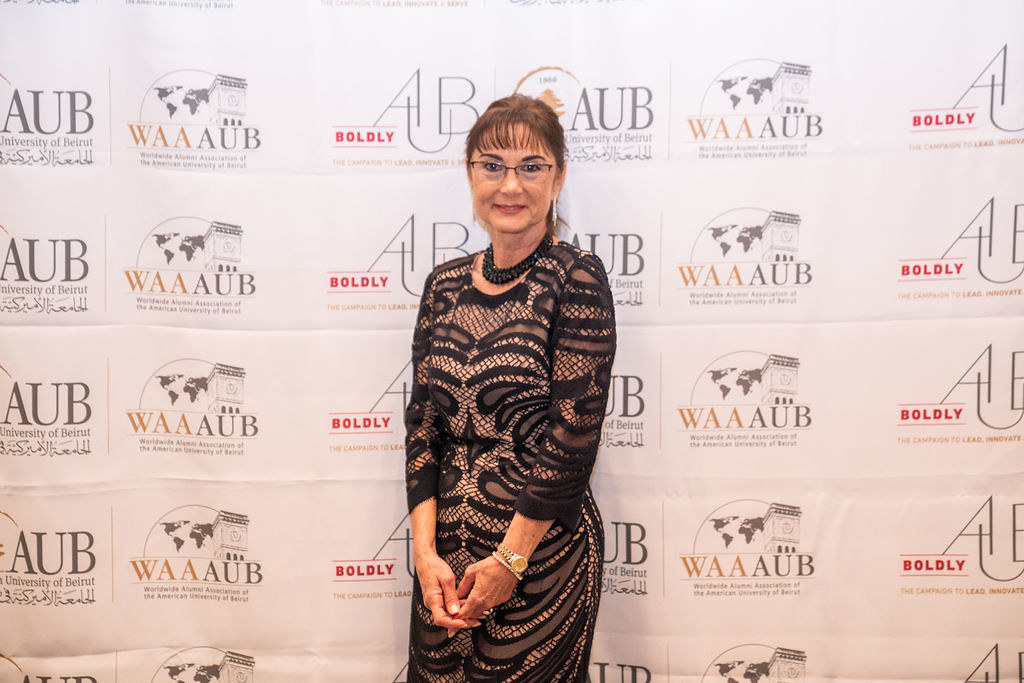This photograph features a woman, likely in her 50s, with brunette hair neatly pulled back and bangs framing her forehead. She is wearing librarian-style glasses and is dressed in a black, lacy dress. She stands with her hands clasped in front of her, wearing a watch and bracelet, and displays a subtle, half smile.

The backdrop features a white background scattered with repeated logos, most prominently the acronyms WAAA and AUB, some of which are stylistically rendered in red and black with brownish accents. These logos are symmetrically arranged in four rows, reminiscent of the promotional backdrops seen at high-profile events like the Oscars.

The image is taken from around thigh-level up, and the woman's central positioning against this event-themed background, possibly affiliated with the University of Beirut, suggests a formal or semi-formal occasion.